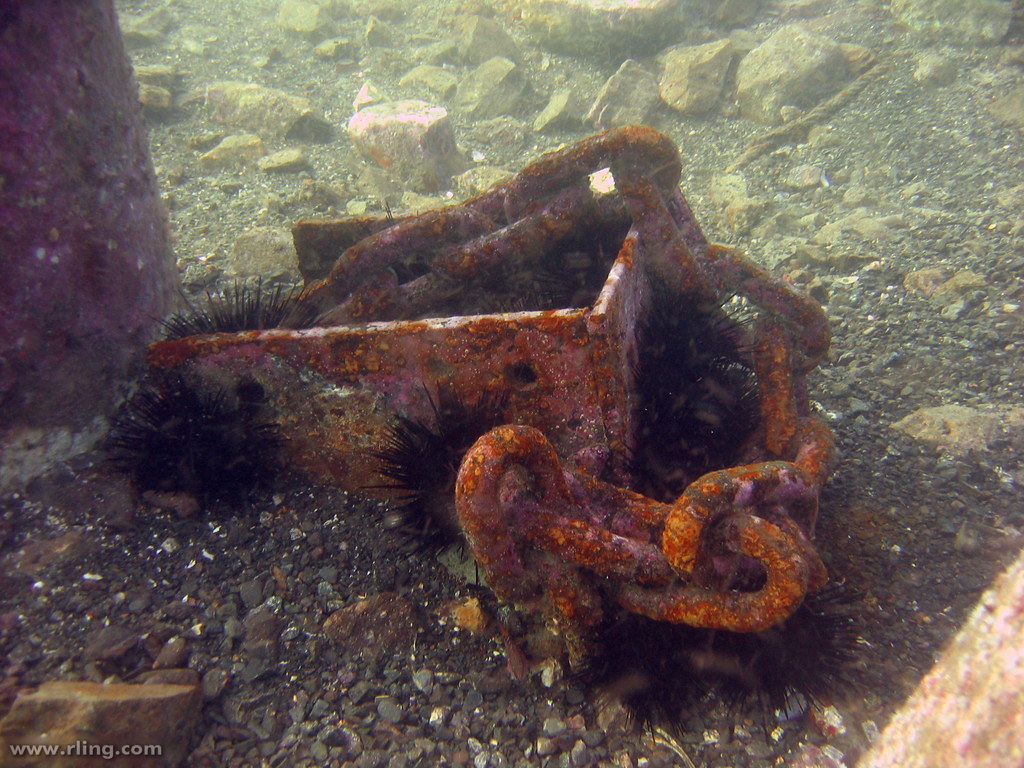The photograph captures what appears to be the bottom of an aquarium or possibly a body of water. The surface is flat and entirely covered with various sizes of gravel and rocks. Dominating the scene is a large, heavily rusted piece of metal with a substantial metal chain coiled around it, resting atop the gravel. Surrounding this iron artifact are several black, spiny sea urchins, their fluffy-looking spines adding an intriguing texture to the image. There are at least five of these sea urchins dispersed around the rusted metal and chain. The background resembles the base of a hill, covered in granite, tiny pebbles, and more gravel, suggesting a natural underwater landscape or a meticulously designed aquarium setup. The composition of the image—with its mixture of rusted metal, ancient chain, and marine life—gives a strong impression of something long-forgotten and reclaimed by nature. In the lower left-hand corner, the image is marked with "www.arling.com," possibly indicating the photographer or source.